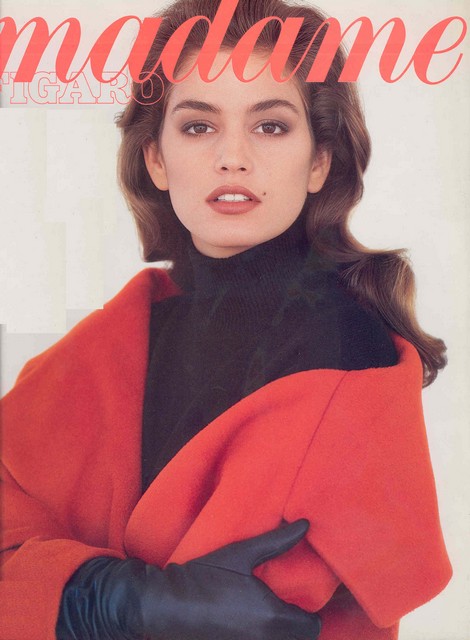The image is a vintage magazine cover featuring a young Cindy Crawford. The magazine title, "Madame," is elegantly written in cursive with orangish-red letters, prominently displayed at the top. Below the title, partially obscured, are the letters "I-G-A-R-O," suggesting the word "Figaro." Cindy Crawford, with her striking beauty, is the sole focus of the cover. She has long, wavy brown hair brushed back, a lighter skin complexion, and a small beauty mark above her lip accentuated by red lipstick. She is dressed in a black turtleneck sweater, draped with a red long-sleeved jacket over her shoulder, and she wears black leather gloves. Her arms are confidently folded as she stands against a white or cream-colored backdrop, illuminated by natural light.